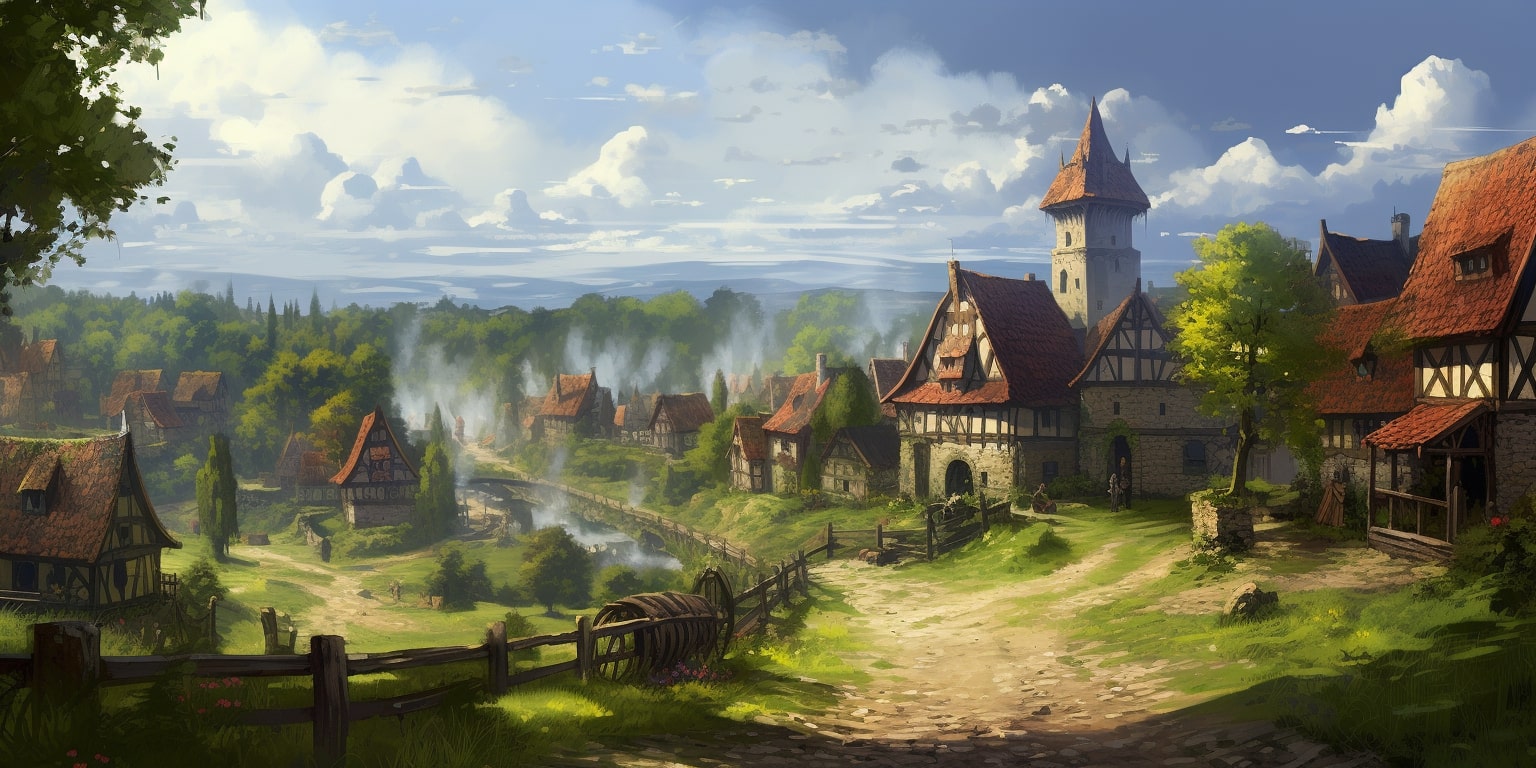The image is a panoramic painting, likely from the 19th century, depicting a sprawling medieval village nestled within a dense forest. The village is characterized by multiple homes on both sides of dirt roads, featuring brown shingle roofs and distinctive architectural elements reminiscent of Norwegian or German styles, with shingles and brick bases. There's a rustic wooden fence with two horizontal beams stretching far into the distance on the left side. A river or creek, possibly a canal, runs through the center, with steam rising along its path, suggesting controlled burning or other activities. Mountains with billowy white clouds hover in the distant background, while patches of blue sky break through, especially in the upper right-hand corner. The trees in the scene are primarily deciduous, interspersed with a few pines, and the overall feel of the painting blends realism with touches of Impressionism.